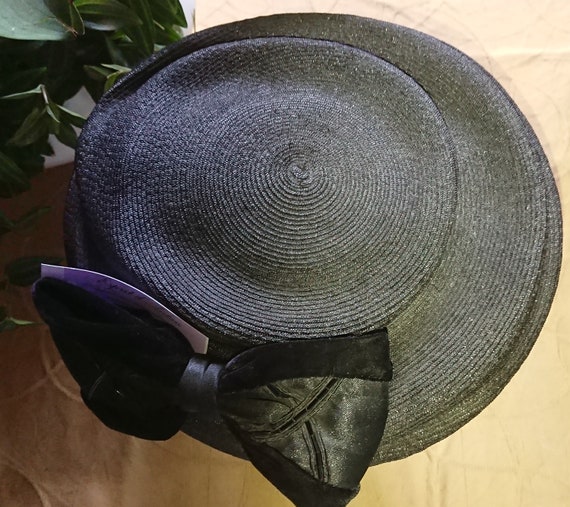The image features a round black hat resting on a yellow-colored surface. The hat has a distinctive design, with concentric circles originating from the center and expanding outward until midway, where the form then drops straight down and flares out again towards the brim. Attached to the bottom left side of the hat is a large black bow, beside which is a pink piece of paper nestled between the bow and the hat. The surface underneath displays varying shades of yellow, with the lightest section in the upper right corner and progressively darker shades, including shadows, in the bottom left corner. In the upper left corner, green leaves from a plant are visible, and there appears to be a white piece of paper or plate holding the plant up. The lighting is more intense on the right side, illuminating the upper portions of the hat and bow while leaving the left side in shadow.